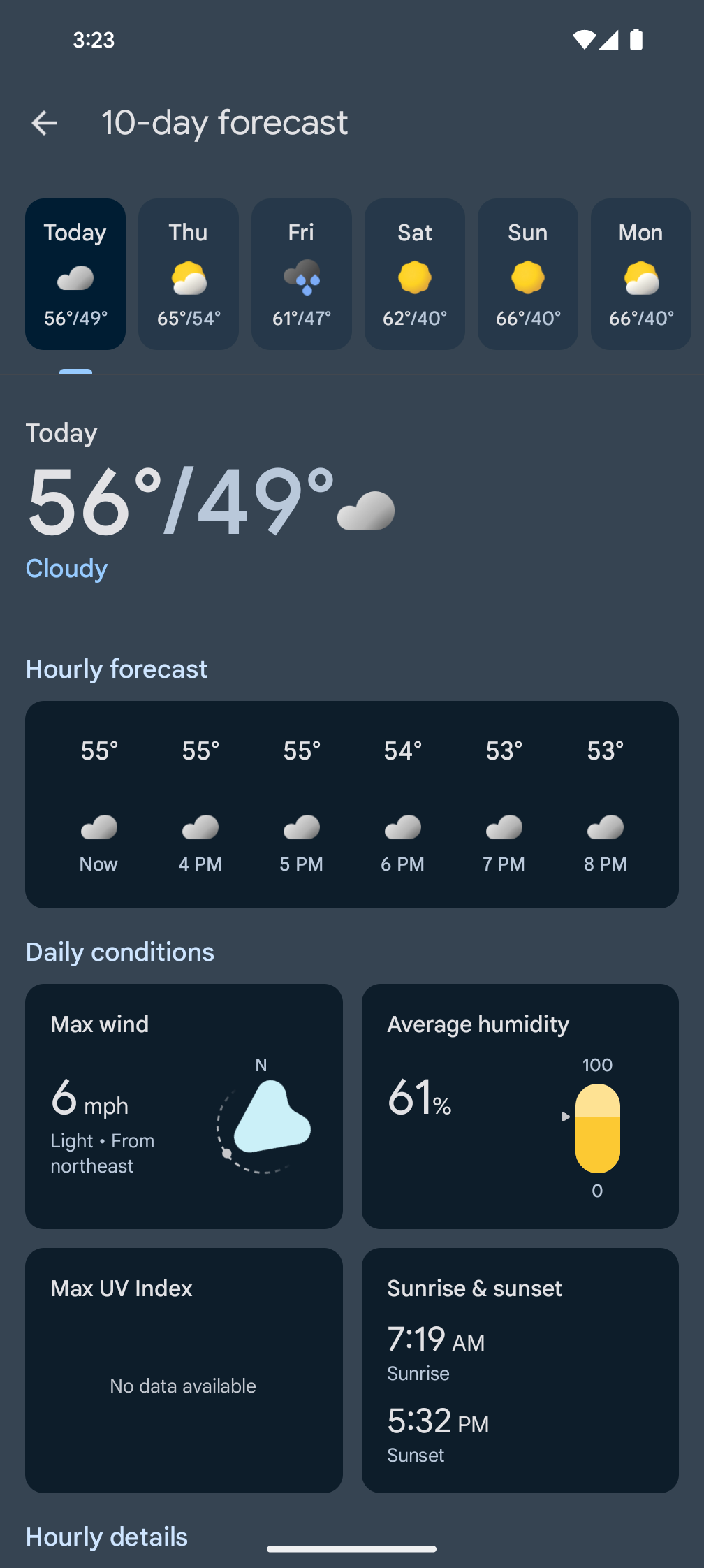Here's a detailed and cleaned-up caption for the image described:

---

The image is a screenshot of a weather forecast displayed on a dark gray background. At the top of the screenshot, icons for time (3:23), Wi-Fi, full signal, and full battery are visible. Below these icons, a left-pointing arrow and the text "10 Day Forecast" are presented, leading into a 6-day weather outlook.

### 10-Day Forecast (Partial)
- **Today**: Cloudy with a high of 56°F and a low of 49°F. Represented by a cloudy icon.
- **Thursday**: Partly cloudy with a high of 65°F and a low of 54°F.
- **Friday**: Rainy with a high of 61°F and a low of 47°F.
- **Saturday**: Sunny with a high of 62°F and a low of 40°F.
- **Sunday**: Sunny with a high of 66°F and a low of 40°F.
- **Monday**: Partly cloudy with a high of 66°F and a low of 40°F.

### Today's Detailed Forecast
- **Temperature**: High of 56°F, low of 49°F. A cloudy icon is accompanied by the word "Cloudy."

### Hourly Forecast
- **3 PM**: 55°F, Cloudy
- **4 PM**: 55°F, Cloudy
- **5 PM**: 55°F, Cloudy
- **6 PM**: 54°F, Cloudy
- **7 PM**: 53°F, Cloudy
- **8 PM**: 53°F, Cloudy

### Daily Conditions
- **Max Wind**: 6 mph from the northeast. An icon depicts wind direction with the letter 'N' at the top.
- **Average Humidity**: 61%, shown with a barometer ranging from 0 to 100.
- **Max UV Index**: No data available.
- **Sunrise and Sunset**: Sunrise at 7:19 AM and sunset at 5:32 PM.

The forecast cuts off below the section labeled "Hourly Details."

---

This caption accurately details the visual elements and weather information presented in the screenshot.